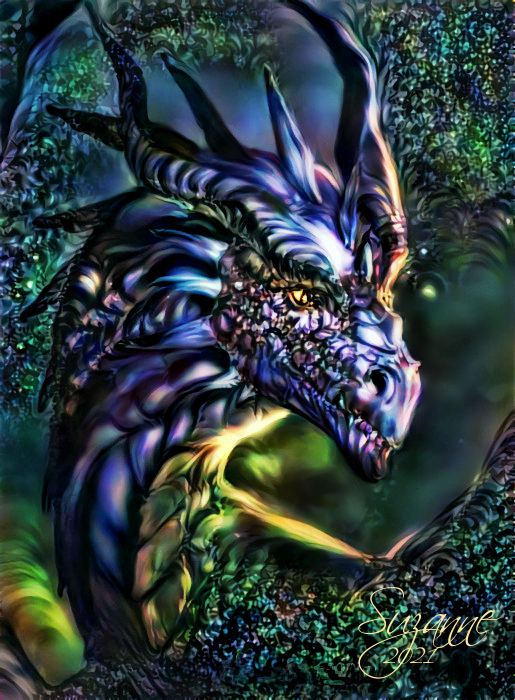This image features an intricate and majestic artistic rendering of a mythological dragon. The dragon, primarily depicted in rich purples with highlights of green, blue, and yellow that blend into a psychedelic, almost stained-glass appearance, gazes to the right. Its bright yellow eyes and the textured, gem-like quality of its scales contribute to its ethereal look. The dragon's head is adorned with two prominent horns and a mohawk-like array of spikes extending backward. The composition blends the dragon harmoniously with its forest-like surroundings, which include leafy, mossy textures, giving the illusion that the creature is emerging from a vibrant, colorful wilderness. At the bottom right of the image, in cursive yellow font, a barely legible signature followed by "2021" completes this captivating digital artwork.